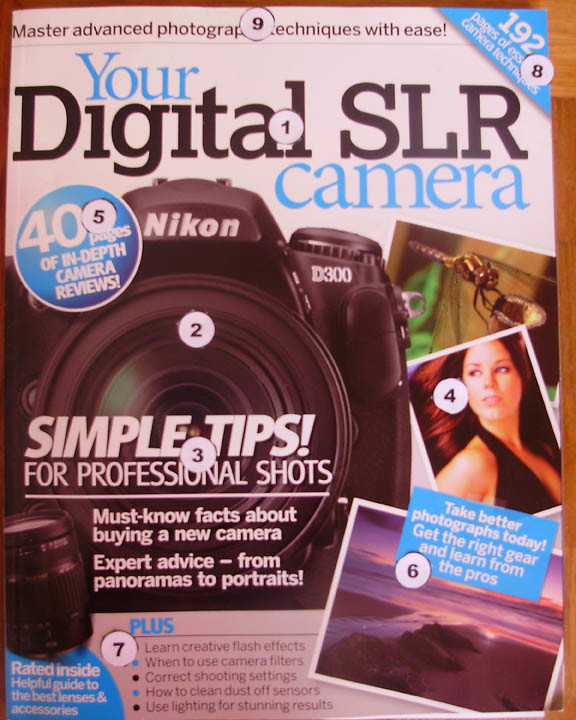The photograph captures the cover of a magazine titled "Your Digital SLR Camera" resting on a wooden coffee table. The magazine prominently features a large image of a Nikon D300 camera, accompanied by an array of other photographs, including a dragonfly, a woman in a black dress, and a beach at sunset. The cover is enriched with numerous headlines and text, boasting "Master Advanced Photography Techniques with Ease" at the top and highlighting "192 Pages of Essential Camera Techniques". Several notable phrases like "Simple Tips for Professional Shots" and "Take Better Photographs Today" are scattered across the cover. The cover appears edited, as indicated by white numerical labels superimposed on various elements: '1' over "Your Digital SLR Camera", '2' over the Nikon camera image, '3' over "Simple Tips", '4' over the woman's photo, '5' over "400 Pages of In-Depth Camera Reviews", '6' over the beach photo, '7' at the bottom near "Learn Creative Flash Effects", '8' over "192 Pages of Essential Camera Techniques", and '9' near "Master Advanced Photography Techniques with Ease". The cover also includes additional smaller text sections, offering advice on topics like "Must Know Facts About Buying a New Camera" and "How to Clean Dust Off Sensors", which makes the cover visually dense and highly detailed.